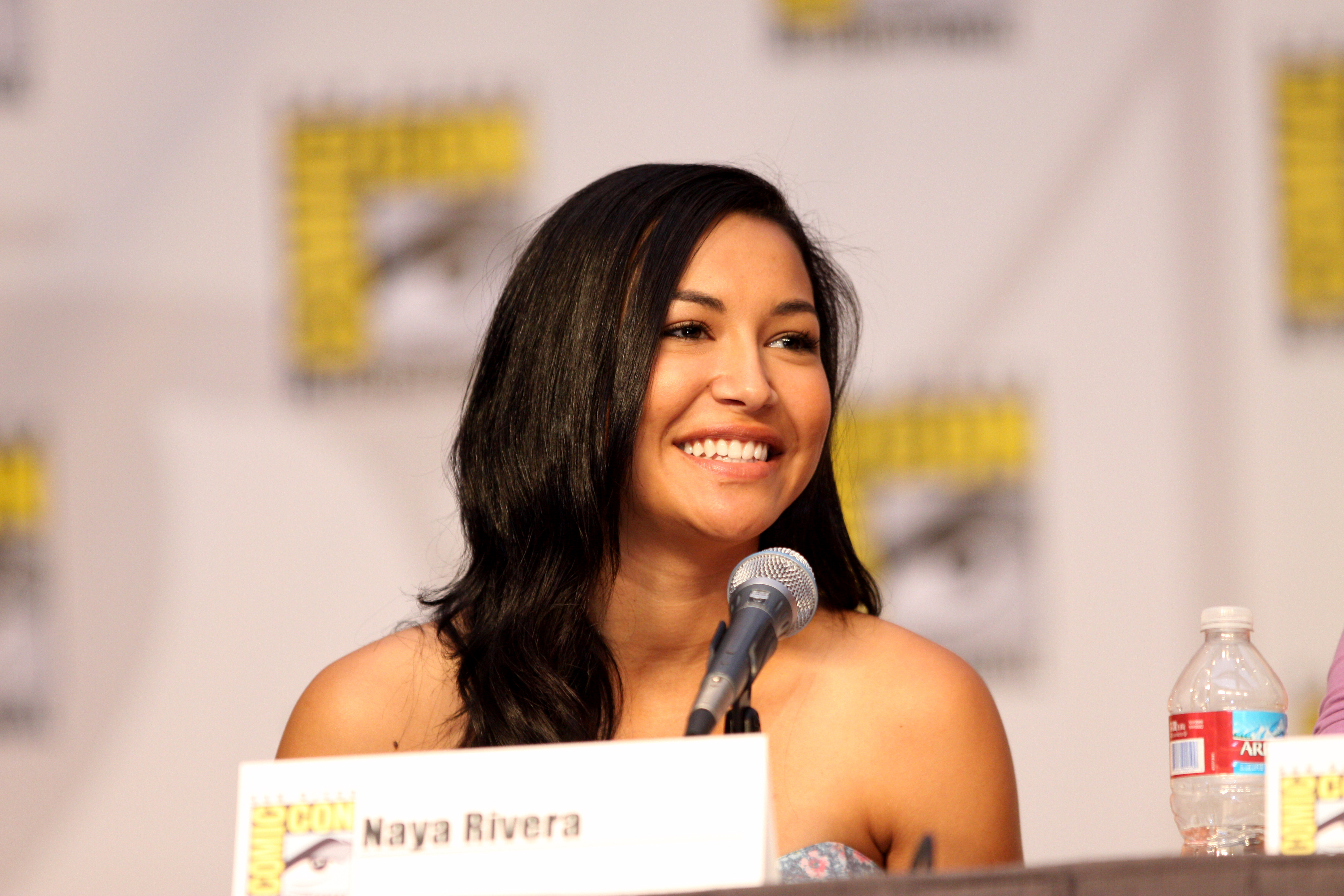In this vibrant photo, the late Naya Rivera from "Glee" is captured at a Comic-Con event, sitting at a long table and engaging with the audience. She is beaming a warm smile, directed at someone off-camera. A microphone is positioned in front of her, suggesting she is answering questions or participating in a discussion. Her black hair, styled in slight waves, gracefully cascades around her chest. In front of her, a name tag reads "Naya Rivera" alongside the Comic-Con logo. To her left (our right) is a water bottle and another Comic-Con name card, with the arm of a fellow panelist in a pink striped outfit just visible. The background features a white banner adorned with blurred, repetitive Comic-Con logos, adding to the immersive atmosphere of the event. Rivera’s demeanor reflects her enjoyment and engagement in the moment, surrounded by the dynamic energy of Comic-Con.